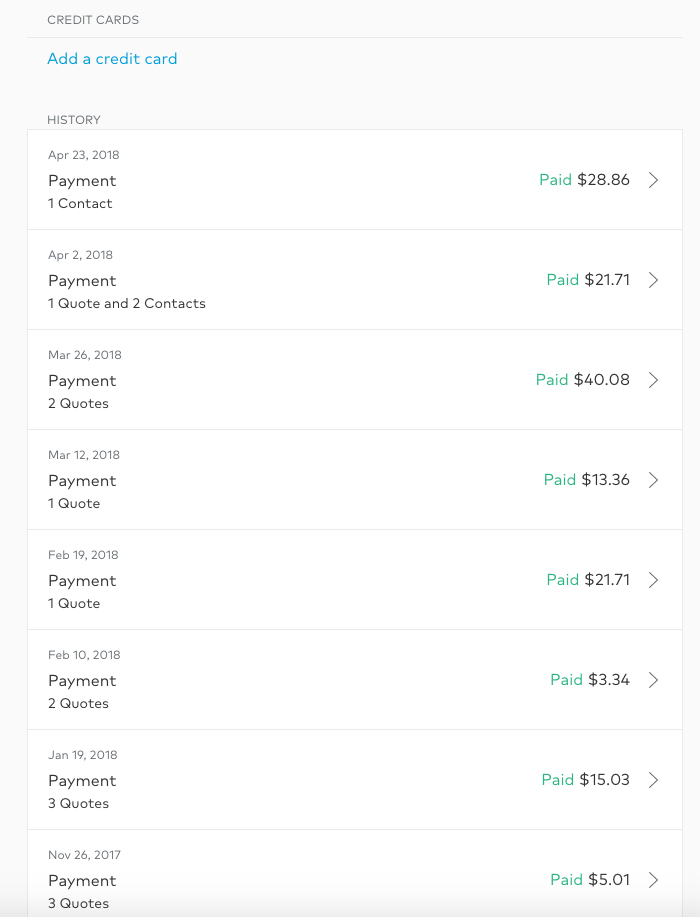This vertical image appears to be a screenshot taken from a smart device. The background is a light to medium gray. At the top, in uppercase letters, there is the heading "CREDIT CARDS" in a grayish color. Beneath this heading is a thin gray line, which separates it from the next section. Below the line, in blue text, it reads "Add a Credit Card." Following this, the word "History" is displayed.

The image features a white box divided into sections by thin gray lines, forming a list of transactions. Each transaction is detailed with the date in gray, the payment description in black, and the status "PAID" in green on the right side, followed by the corresponding amount in black. For instance:

1. April 23rd, 2018: Payment one contact, PAID, $28.86
2. April 2nd, 2018: Payment one quote and two contacts, PAID, $21.71
3. March 26th, 2018: Payment two quotes, PAID, $40.08
4. March 12th, 2018: Payment one quote, PAID, $13.36
5. February 19th, 2018: Payment one quote, PAID, $21.71
6. February 10th, 2018: Payment two quotes, PAID, $3.34

This pattern continues for two more transactions, following the same format.